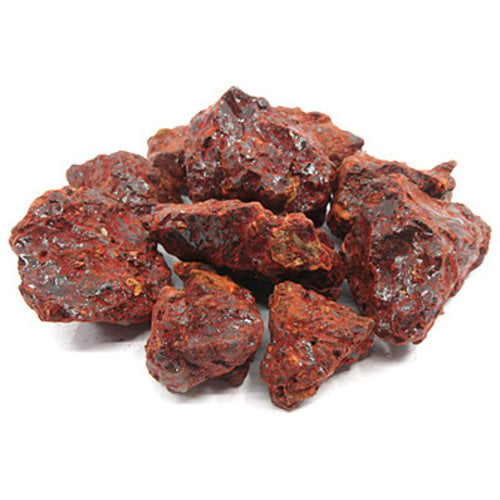The image showcases a group of about eight irregularly shaped, reddish-brown rocks arranged in a circular pattern on a white background. The circular formation consists of six rocks around the perimeter and two in the center. Each rock exhibits various shades of reddish-brown with additional hints of gray, white, orange, and a burnt yellow. Shadows under some of the rocks add depth to the scene. The rocks are different sizes; the one in the very front on the left is rounder, while the adjacent one to the right is more triangular. Larger rocks occupy the outer circle, with a medium-sized rock standing upright in the center. Their composition and arrangement suggest they might be red lava rocks, potentially laid out for a photo shoot, such as for a magazine or a museum exhibit.